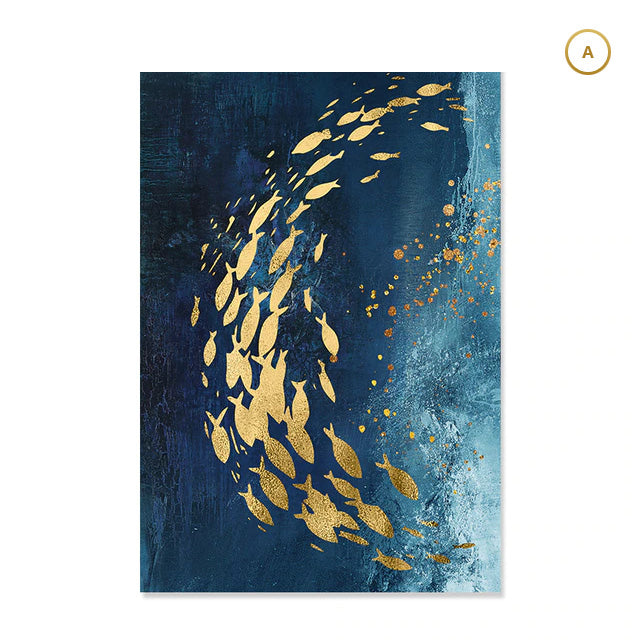This painted artwork depicts a mesmerizing school of gold fish swimming in a graceful, swirling pattern. The background transitions dramatically from deep, dark blues in the top left to much lighter blues and almost white in the bottom right, creating a captivating gradient effect. The fish, rendered as gold silhouettes with subtle darker gold speckles, lack fine details, giving them a stenciled appearance. They start from the top right, curve towards the left, and then descend downwards before arcing back to the right. The overall composition gives a sense of fluid motion and harmony as the fish navigate through the water. Interspersed among them are numerous tiny gold dots, suggestive of bubbles. Additionally, a striking gold circle with the letter 'A' in gold is present at the very top right, adding a unique focal detail. The blend of colors and the dynamic arrangement of the uniform-sized fish contribute to the painting's ethereal and tranquil quality.